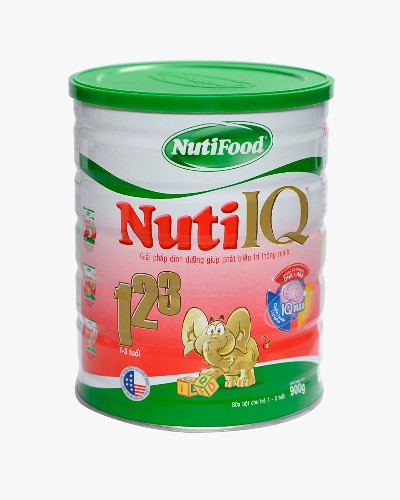This is a photograph of a can of Nutri-IQ baby food, taken against a plain white background, likely from a website or catalog. The can is topped with a green plastic lid. It features a colorful label, which predominantly shows the Nutri-Food and Nutri-IQ brands, with "NewT IQ" prominently written in red and brown text. The label's design includes a whimsical yellow elephant in the center, playing with toy ABC blocks, symbolizing early learning. Additionally, there are small icons to the right, including an image of a brain, likely emphasizing the product's cognitive benefits. The background of the label transitions from light pink at the top to a deep red at the bottom, where the green ground layer depicts the surface the elephant is standing on. The bottom left corner displays a USA flag, while "900 grams" is clearly indicated at the bottom right.